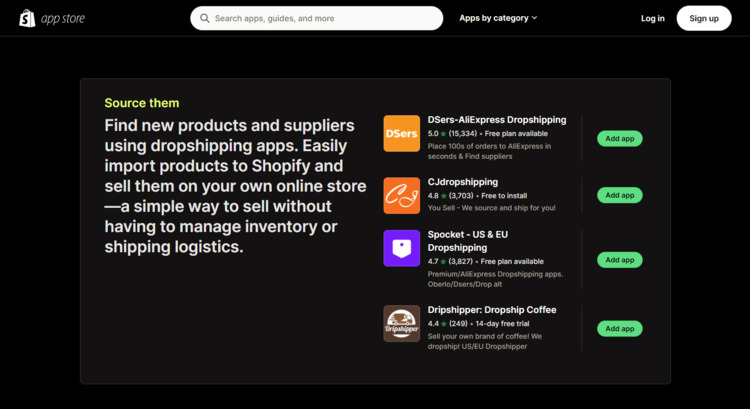Detailed Caption: 

The image is a screenshot of the Shopify app with a sleek black background. Prominently located in the upper left-hand corner is the distinctive Shopify logo, featuring a white shopping bag icon with a black "S" in the center. Adjacent to the logo, the text "App Store" is clearly displayed. 

Centrally positioned at the top of the page is a search bar, flanked on the right by a "Apps by Category" drop-down menu. At the far right corner, two options are available: a "Login" link and a contrasting white "Sign Up" button.

Dominating the center of the page is a square section, slightly lighter than the rest of the background, providing a visual contrast. In the upper left corner of this section, bold yellow text reads "Source Them." Below, white text elaborates: "Find new products and suppliers using dropshipping apps. Easily import products to Shopify and sell them on your own online store - a simple way to sell without having to manage inventory or shipping logistics."

This description is followed by a list of four dropshipping stores, arranged vertically down the page. The first store listed is "De-Essers, Ally Express Dropshipping." The second is labeled "CJ Dropshipping." Next is "Sprocket US and EU Dropshipping." The final store icon is for "Drip Shipper Dropship Coffee." 

The overall layout and cohesive design elements make this a user-friendly and visually appealing section of the Shopify app, focused on helping users streamline their e-commerce processes through dropshipping.